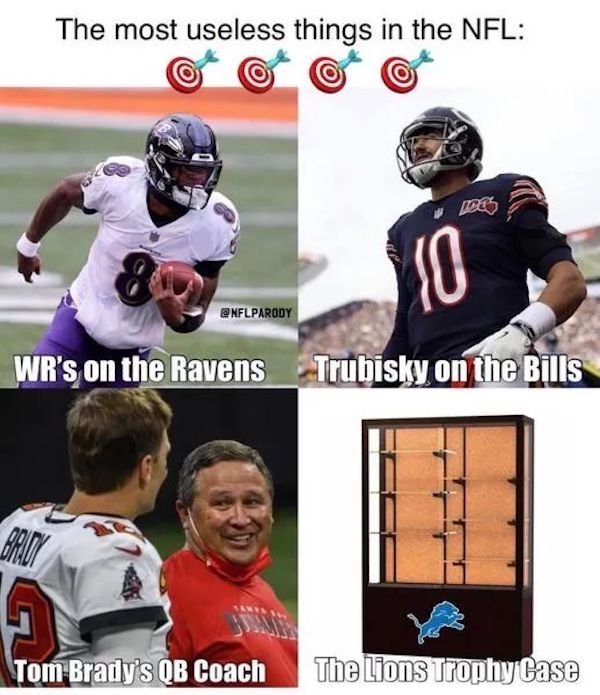This meme features a satirical critique titled "The Most Useless Things in the NFL" illustrated in a window-pane style with four distinct images. The top-left panel depicts a Baltimore Ravens wide receiver, dressed in a black helmet, white jersey, and purple pants, running with a football. The caption reads "WR's on the Ravens." The top-right panel features Mitch Trubisky in a black Chicago Bears jersey with orange stripes, labeled "Trubisky on the Bills." The bottom-left panel shows Tom Brady in a Tampa Bay Buccaneers uniform, alongside his coach in an orange Buccaneers sweatshirt, captioned "Tom Brady's QB Coach." The bottom-right panel displays an empty black wooden trophy case adorned with a blue Detroit Lions logo, labeled "The Lions' Trophy Case." The overall color palette includes black, white, red, blue, purple, orange, and brown. The meme is structured with humor and irony, using these visual elements and captions to satirically comment on perceived inefficiencies within the NFL.